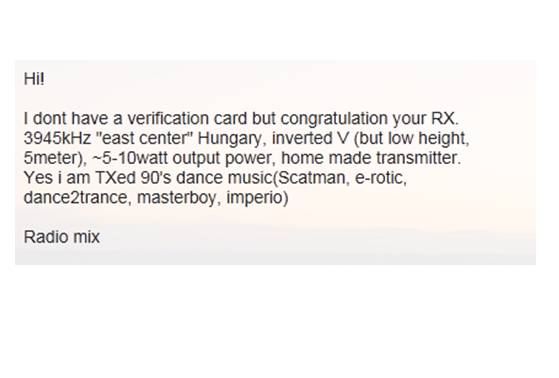This image features a rectangular block of text in black print on a slightly off-white background with a subtle pinkish tint. The text appears to be a screenshot of an email or a message. It reads as follows: 

"Hi! I don't have a verification card, but congratulations, your RX 3945 kHz 'East Center,' Hungary, with an inverted V antenna at a low height of 5 meters. The transmitter has an output power of 5 to 10 watts and is homemade. Yes, I am TXing 90s dance music including Scatman, Erotic, Dance to Trance, Masterboy, and Imperio. Radio mix."

The message seems to detail specifications of a radio transmission setup and mentions a fondness for 90s dance music, celebrating the receipt or operation of certain radio equipment.